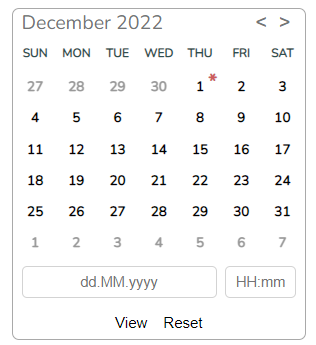This screenshot captures a digital calendar interface displaying the entire month of December 2022. The calendar is presented on a white background with black font, providing a clean and clear view. December 2022 begins on a Thursday, and dates from the previous month—November 27th through the 30th—are displayed in a lighter gray. 

The calendar layout starts from Sunday on the left and progresses towards Saturday on the right. A notable detail is the red asterisk next to December 1st, which stands out against the otherwise monochromatic scheme. The month spans four weeks, concluding on Saturday, December 31st, followed by the beginning of January’s days faintly visible at the bottom.

In the top right corner, navigation arrows are available, allowing users to switch between November and January. Below the calendar grid, a formatting box is visible, displaying a placeholder text “dayday.monthmonth.yearyearyearyear,” indicating the editable format for date entries. Next to this, there is an input field labeled "HHMM" for hours and minutes specification. At the very bottom, there are "View" and "Reset" buttons for user interaction.